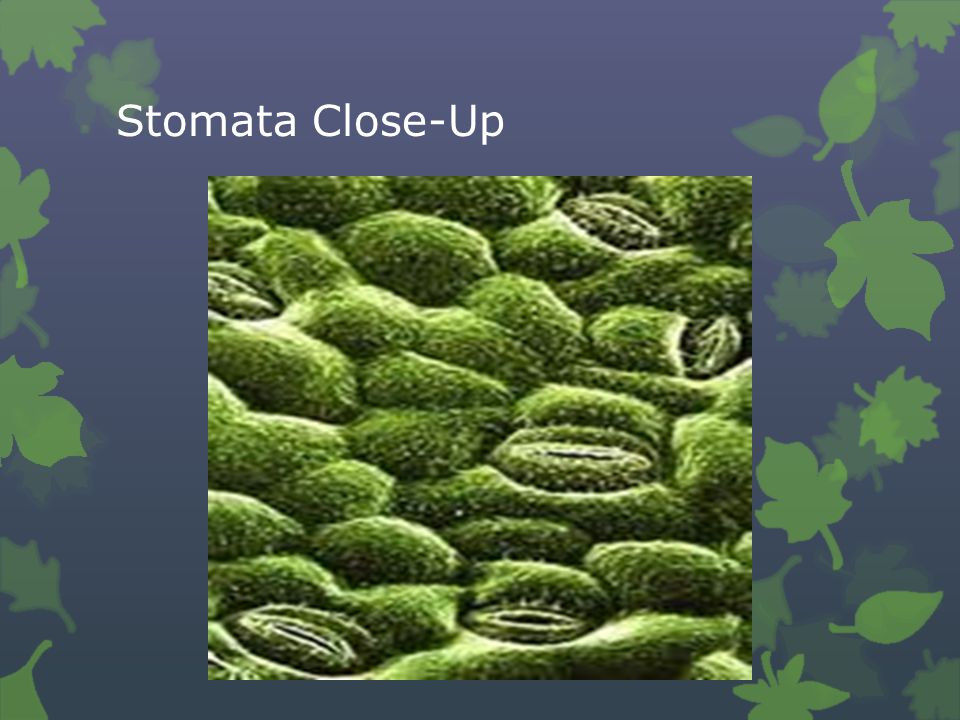The image, titled "Stomata Close-up," seems to be a very zoomed-in and somewhat grainy photograph, possibly taken using a microscope or a scanning electron microscope. The picture is framed with a purplish-blue border, accompanied by green leaves on both the left and right sides, suggesting a natural, digitally enhanced design. At the center of the image lies the focal subject: a colorized photograph of stomata, featuring numerous green, bum-like structures of various sizes that resemble round stones covered in green moss or tiny leaves. Some of these structures, especially those near the middle, exhibit discernible horizontal openings. The top left corner of the image prominently displays the text "stomata close-up" in white. The overall appearance and composition suggest that this image might be part of a presentation, like a slide in a PowerPoint deck, featuring different shades of green, yellow, white, and gray.